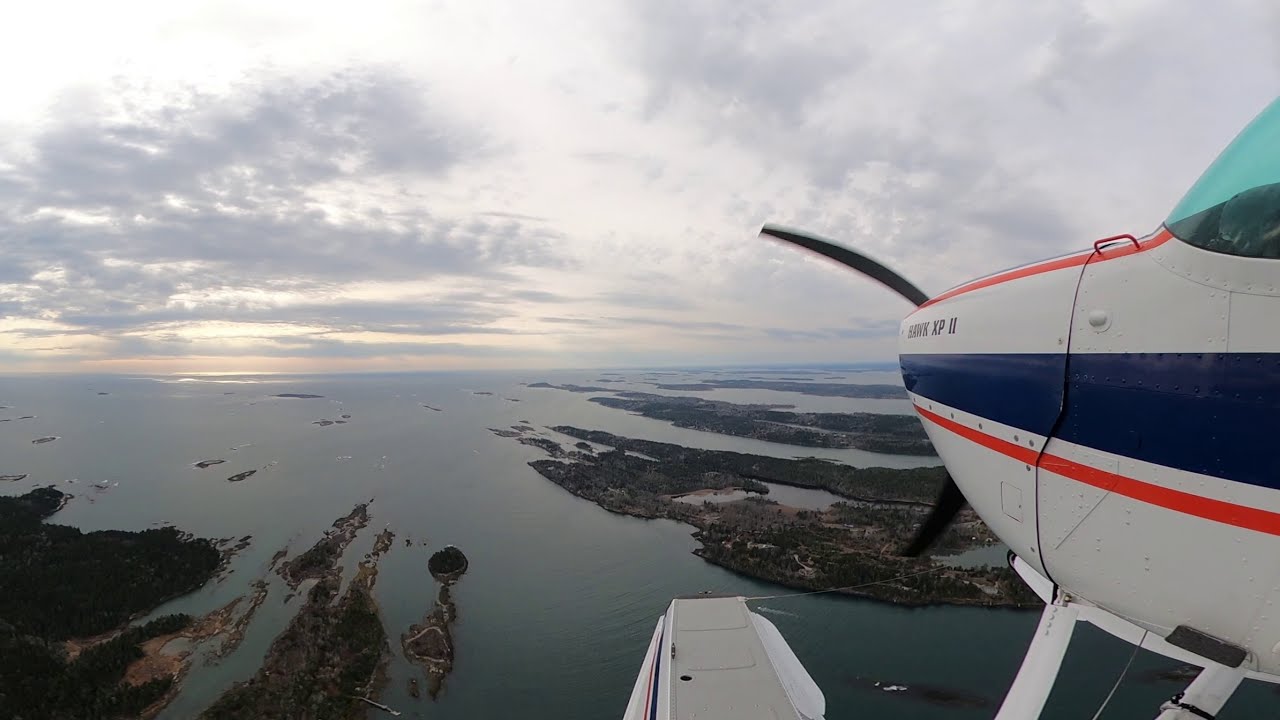This aerial image, likely taken from a small plane or helicopter, captures a captivating scene of nature as viewed from the sky. Prominently featured is the nose of a white aircraft adorned with blue stripes in the middle and red stripes above and below, with 'Hawks XP2' inscribed along the side. The black propeller is partially visible. Below, the scenery consists of an expansive body of water interspersed with unique land formations, resembling islands or channels. The land, appearing as small, distinct strips, shows minimal human development, enhancing the natural beauty of the scene. The sky is filled with clouds, and the sun is setting on the horizon, casting a dusky glow over the landscape. The image is serene and isolated, with no visible signs of human or wildlife activity, apart from the unseen pilot of the aircraft.